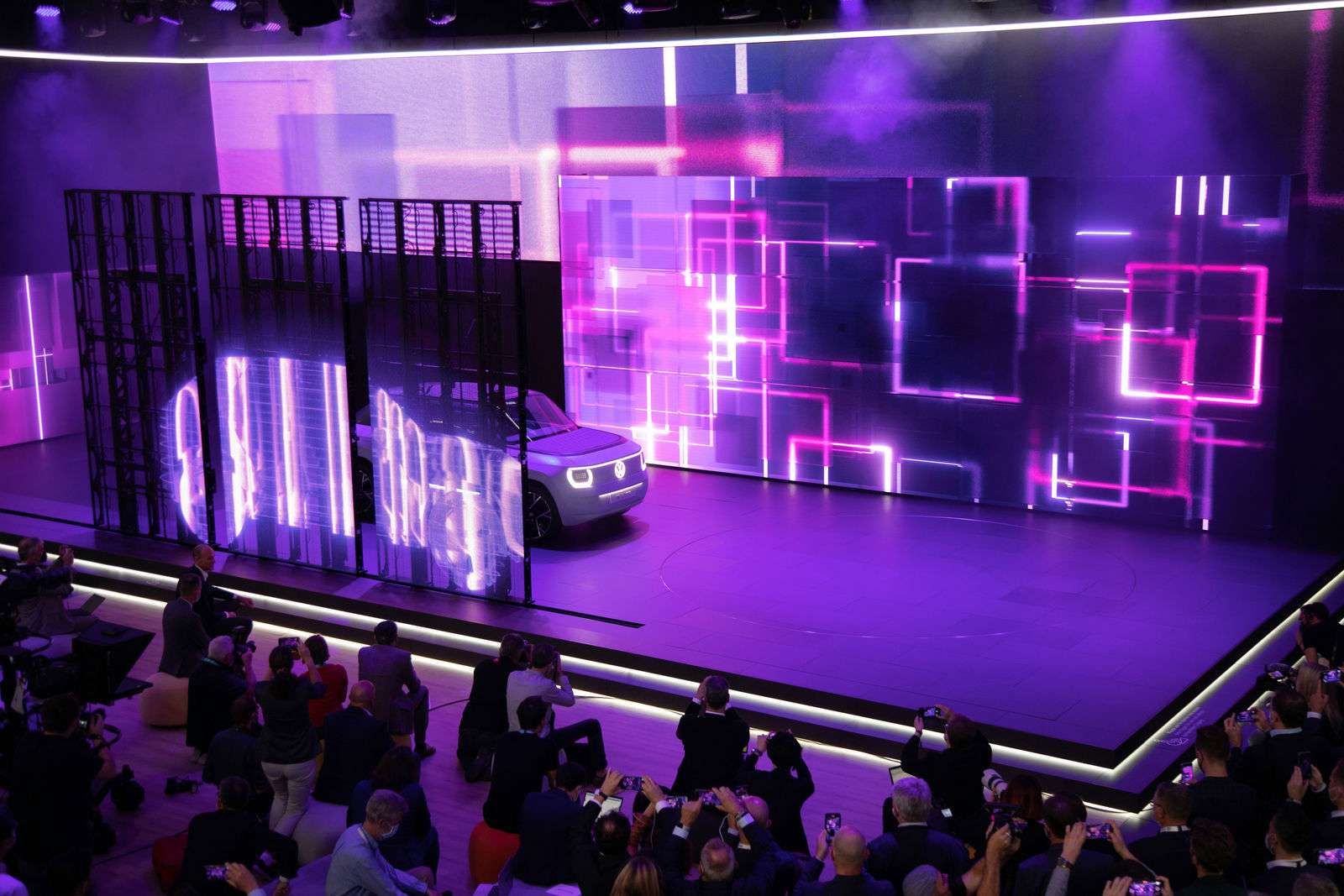In this detailed color photograph, a sleek white car with illuminated headlights is prominently displayed on a stage awash in purple and black hues. The stage is two steps high, each edge highlighted by white lights, and is surrounded by a diverse audience, many of whom are formally dressed and seated on cushioned chairs. Behind the car, a striking backdrop features an array of neon geometric shapes, predominantly squares and rectangles, in white and various shades of purple, pink, and blue. These shapes overlap and create a dynamic visual effect, illuminated by strategically placed lights. A large panel with a metal frame and wooden cross beams stands in front of the car, displaying a projected image of the vehicle in white light. The atmosphere is vibrant and bustling, with several attendees holding up smartphones to capture the scene, while a noticeable large television camera on the left records the event.